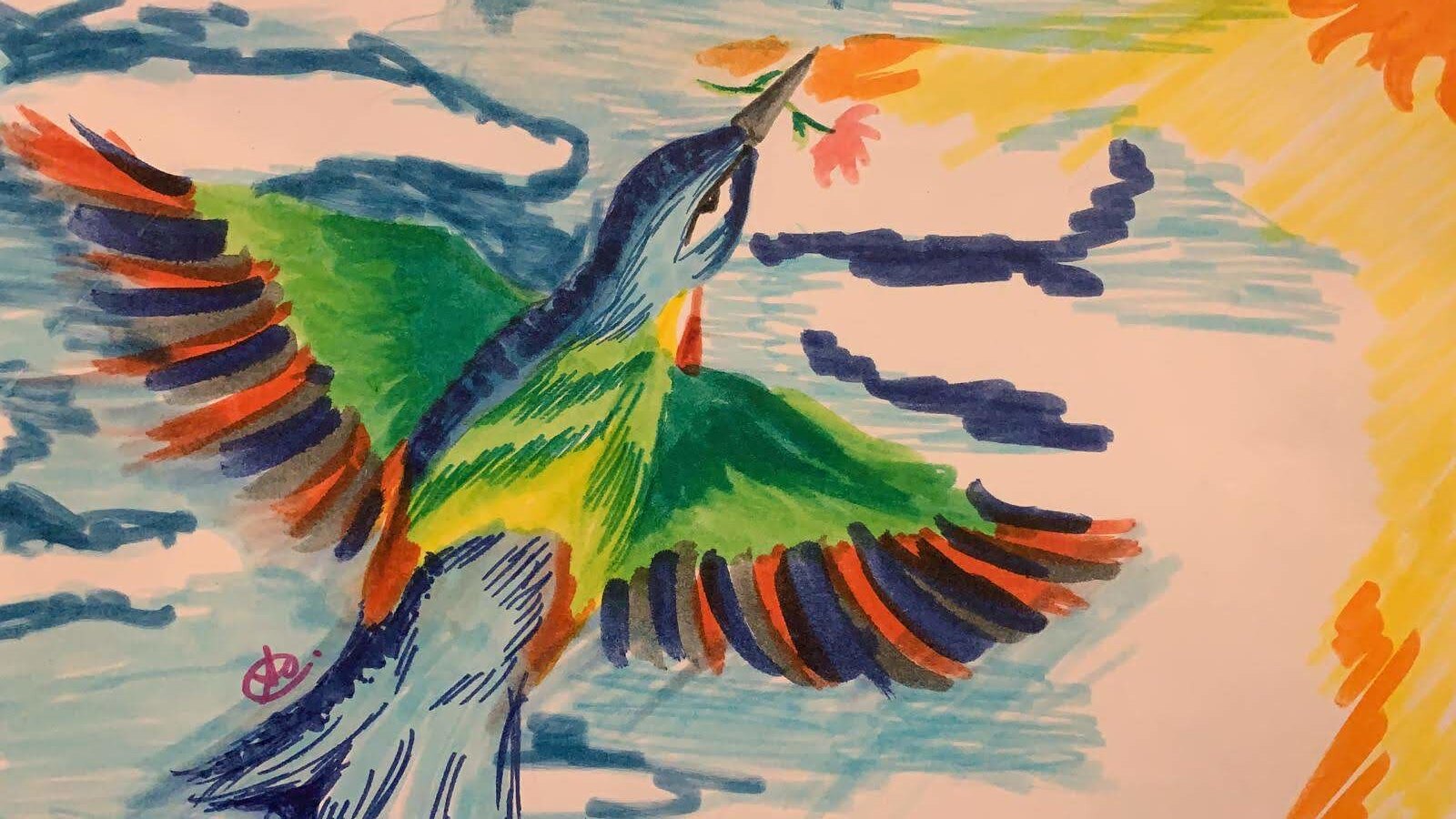This vibrant marker drawing features the artist's signature enclosed in a pink circle, located in the lower-left corner, indicative of a personal touch. The focal point of the artwork is a beautiful bird mid-flight, with its body angled upward and its head slightly turned to the right, capturing a sense of graceful motion. In its beak, it delicately holds a single pink flower, adding an element of charm and tenderness. The bird's body is primarily blue, complemented by striking green wings that taper into blue and orange tips. This colorful avian figure is set against a dynamic background; the right side of the illustration is awash with warm hues of yellow and orange, possibly suggesting the presence of sunlight. The rest of the sky is painted in light blue shades, interspersed with dark blue-outlined clouds, creating an enchanting and lively scene.